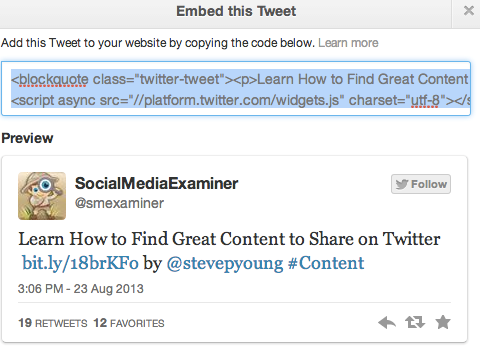This is an image capture of a digital interface, either from a computer or a phone screen, showcasing the Twitter embed feature. At the top of the screen, there is a gray rectangle containing the text "Embed this Tweet." Below this header, on a white background, black text instructs users to "Add this Tweet to your website by copying the code below." Directly beneath this instruction, a gray link labeled "Learn more" is provided for further information.

Within the main section of the display, there is a prominent white rectangle outlined in blue, containing embedded HTML code. The code snippet includes a blockquote with a class attribute set to "twitter-tweet," and text such as “Learn how to find great content,” along with various HTML and UTF-8 elements underlined in dotted red. This indicates syntax or format alerts.

The image also features a preview section labeled "Preview" in black text. Adjacent to this text, there is an icon representing a cartoon character wearing a hat, indicating the Social Media Examiner profile. Directly beneath the icon, the text reads, "Learn how to find great content to share on Twitter," followed by a shortened Bitly URL link for additional content. The embedded tweet showcases engagement statistics, noting "19 Retweets" and "12 Favorites."